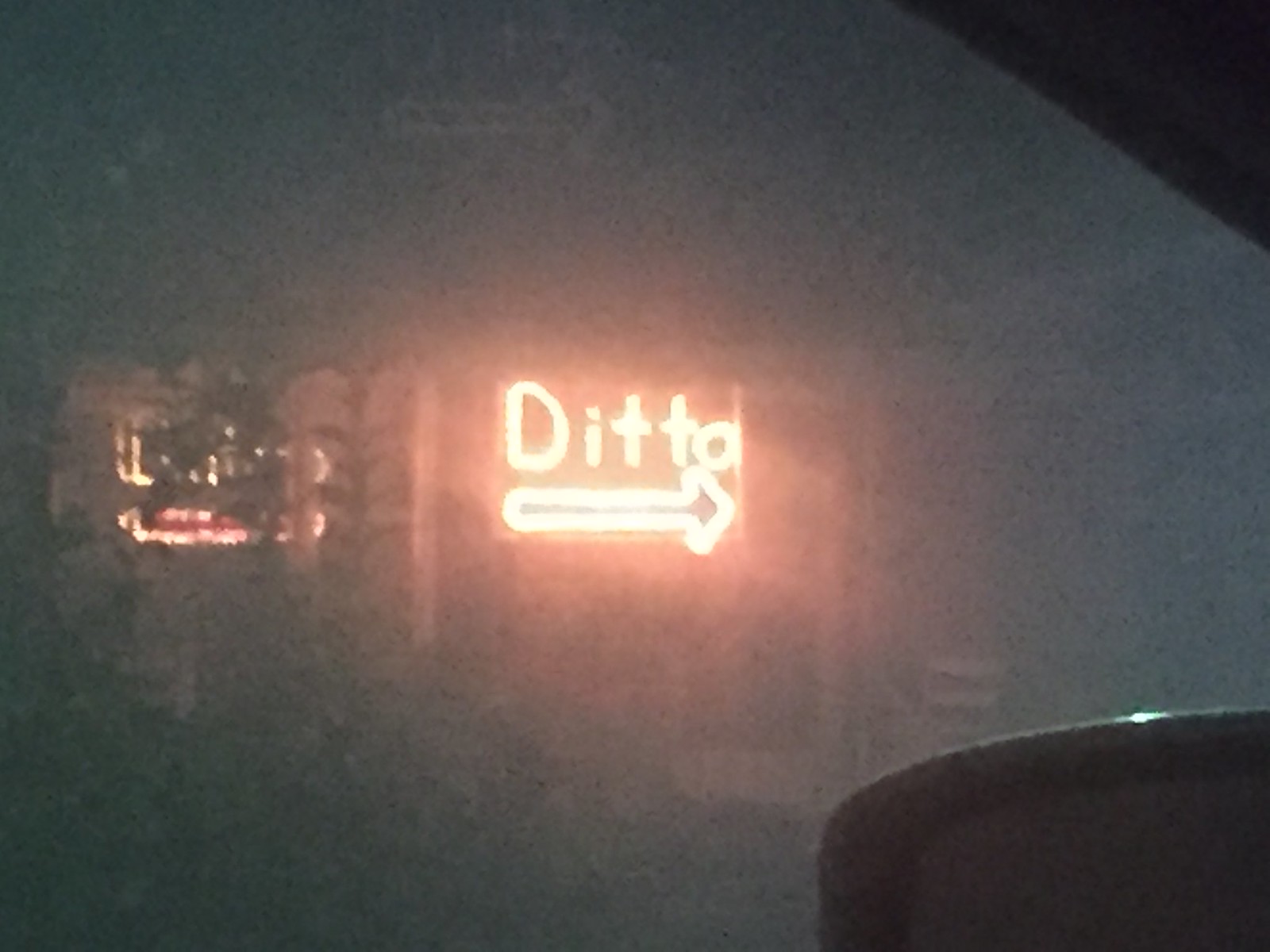The slightly rectangular and horizontally oriented image is grainy and blurry, portraying a view from a driver's side window. In the lower right corner, the upper left portion of the rearview mirror is visible, while the upper right corner captures the angle of the window frame slanting leftwards. Through the window, a storefront or shop is discernible. The storefront's visibility is compromised by the graininess, but a prominent neon sign reading "Ditto" is attached, with an arrow beneath it also in neon, pointing to the right side of the frame. The neon sign contributes to the image's distortion, adding a vivid yet blurry glow to the scene.